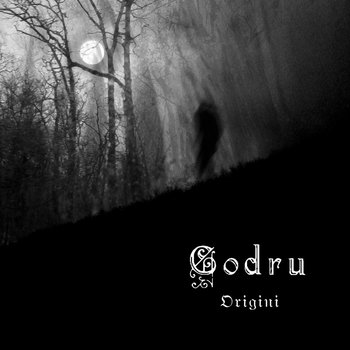The image presents a haunting and eerie night scene rendered in stark black and white. A silhouetted, possibly hunched figure, ambiguous in gender but seemingly adult, is captured descending a slanted, completely black hill. This dark expanse occupies the bottom half of the photo, giving way to an enigmatic landscape above. Bare trees, suggesting a winter setting, stretch across the scene, partially obscured by a thick blanket of mist or fog. The moon, full and luminous, peeks through the branches, casting a faint light that contrasts with the pervasive darkness. Superimposed on the black hill is the text "Godru Oregini," styled in an old-fashioned font, amplifying the unsettling atmosphere. The overall composition, with its shadowy figure, misty surroundings, and antique text, evokes a chilling, thriller-like vibe.